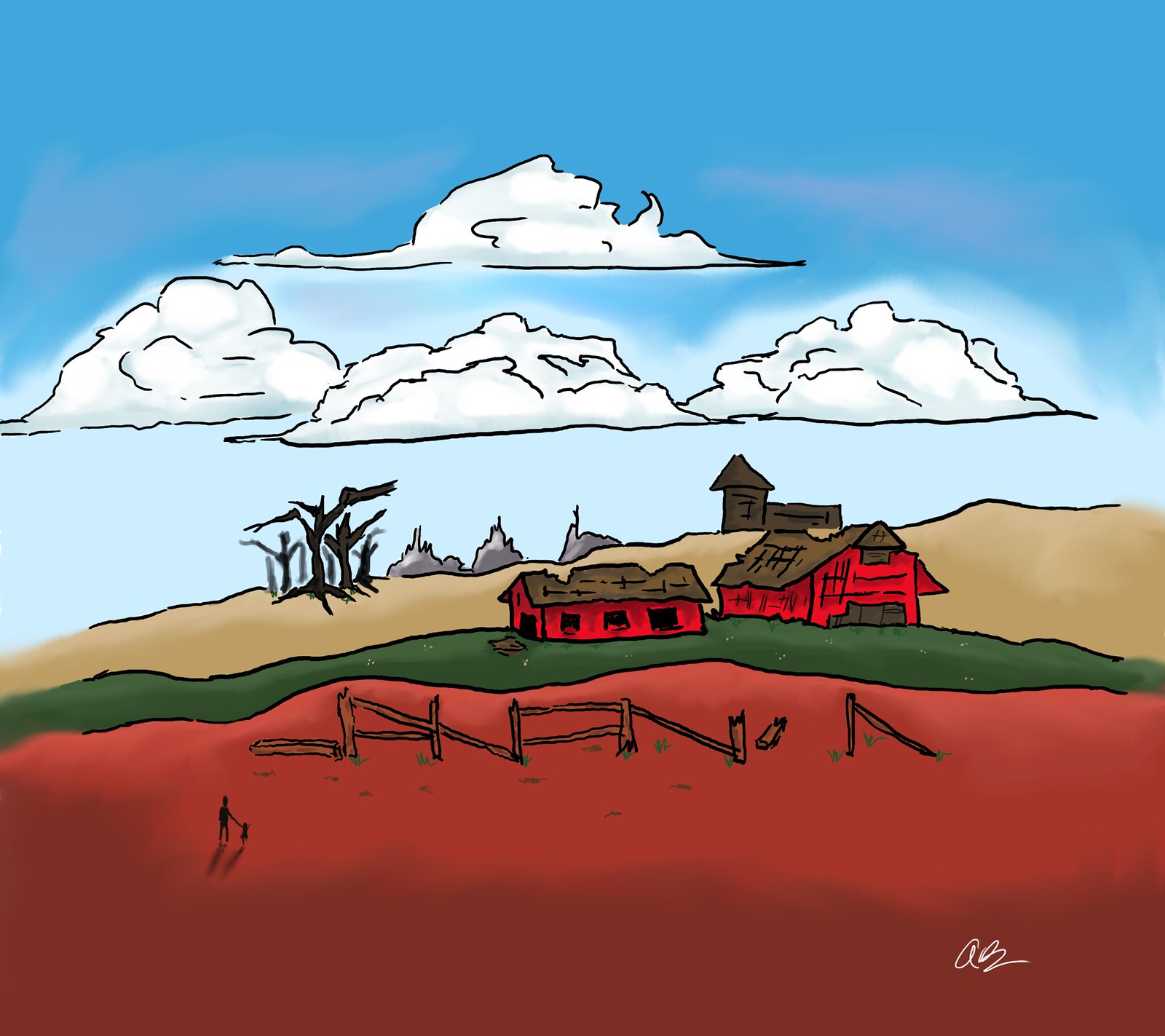The image showcases a vibrant scene under a clear blue sky adorned with scattered white clouds. Beneath the sky, a lighter blue gradient transitions into the horizon. In the foreground, a gently rolling hill composed of golden-brown earth is dotted with several striking features. 

To the left, tall, dark silhouettes of trees stand prominently. Moving towards the center-right, there's a distinct brown building with a conical roof situated on the hill. Behind this building, another structure with grey features can be partially seen. Adjacent to the brown building, a series of red buildings with black windows and wooden rooftops are positioned, adding a splash of color to the scene. Farther right, more red buildings with similar architectural traits extend the vibrant motif.

On the ground level, the scene is grounded by extensive red flooring, creating a contrasting base. In the midst of this setting, a person is seen standing and holding another person's hand, adding a touch of human warmth and connection to the landscape. Intermingled through the lower section of the image, there are scattered fragments of wood, suggesting an area under construction or decay. This detailed composition brilliantly captures a harmonious blend of natural and architectural elements, with human presence adding life to the picturesque scenery.